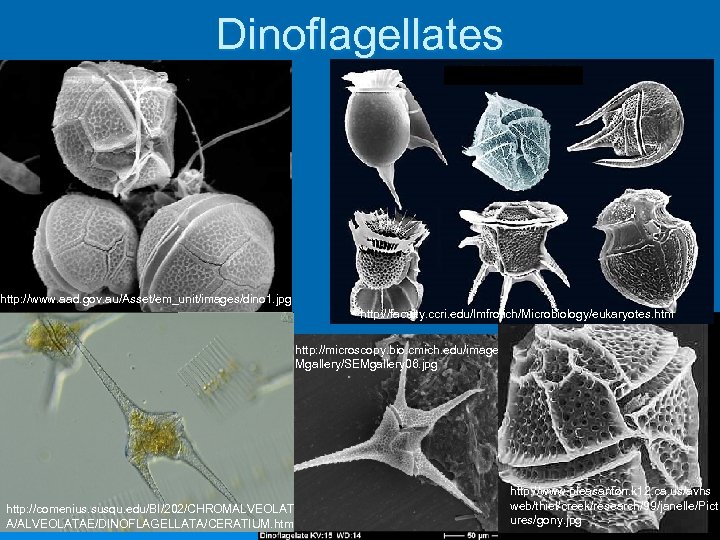The image is a digital slide presentation titled "Dinoflagellates" with the word displayed prominently at the top in white text on a blue background. Below the title, the slide features five highly magnified black and white microscopic images of dinoflagellates, showcasing various types of flagella and cellular structures. A couple of the images have added coloration; one image has a light blue tint, and another shows a light gold center. Each image includes a credit line with tiny white text providing URLs such as http://www.aad.gov.au, http://faculty.ccri.edu, and http://cominius.susqu.edu/bi/202/chromovoltae/dinoflagellates_seridium.htm. The presentation is scientific in nature, illustrating the microscopic detail and complexity of these eukaryotic organisms.